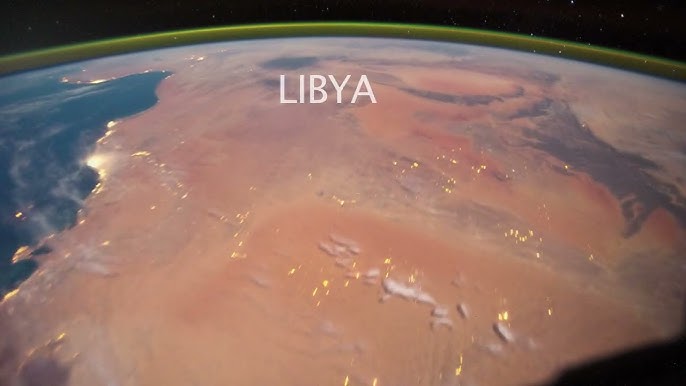This intricately detailed image appears to be a high-altitude or outer space view of Earth, centering on a pink, glossy terrain that somewhat resembles jello with a smooth, shiny surface. This section is labeled "LIBYA" in large capital white letters. The image also features a prominent green outline defining the region. To the left, there's a depiction of deep blue water, possibly an ocean, embellished with white, cloud-like formations. Interspersed throughout the peach or pink-hued landmass are speckles of gold, likely light reflections. The top portion of the image curves, suggesting a planet-like perspective, transitioning into a black expanse mimicking space, dotted with star-like white spots. Additionally, a significant circle on the left side appears subtly illuminated. Overall, the image merges elements of an extraterrestrial view and abstract art.